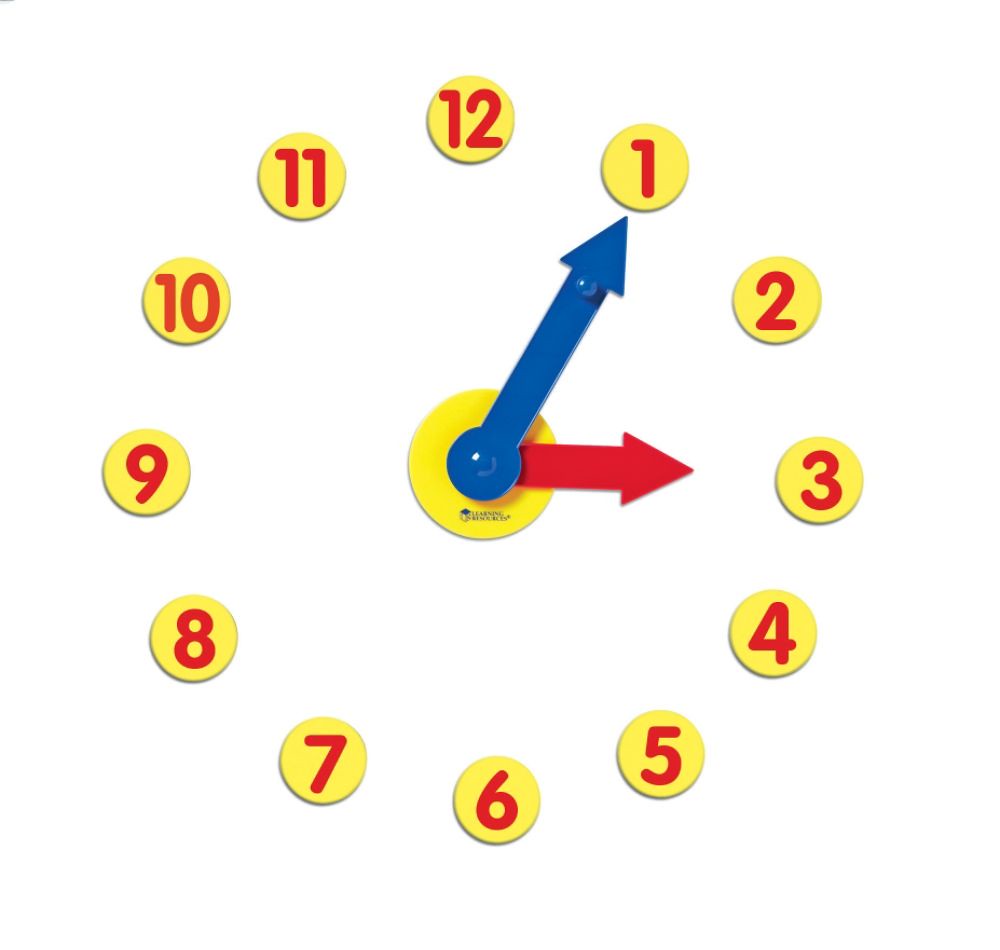The image features a unique clock displayed against an all-white background. Unlike traditional clocks, this one lacks a face or housing. Instead, it comprises a series of yellow discs arranged in a circle, each containing a red number from 1 to 12, mimicking the arrangement of a standard clock. The 12 is positioned at the top, forming a recognizable clock shape. At the center of this arrangement is a larger yellow disc, which serves as the base for the clock hands. The clock hands include a short red arrow pointing at 3 and a longer blue arrow pointing at 1, indicating the hours and minutes, respectively. This central disc also bears a logo or writing, presumably from the manufacturer 'Learning Resources,' suggesting it may be a learning tool designed to teach time-telling skills.